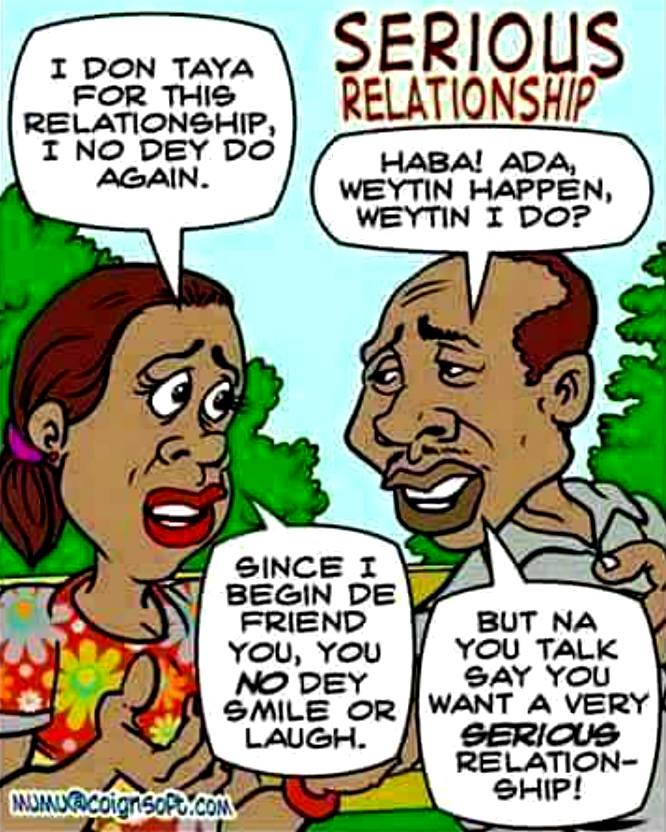The image is a colorful cartoon featuring an African American couple in a park setting with trees and a sky in the background. The woman on the left has brown hair pulled back with a purple tie, wears bright red lipstick, and is dressed in a floral shirt adorned with red, yellow, white, and blue flowers. Her hands are raised as she speaks. The man on the right, with a receding hairline, is wearing a blue collared shirt and faces the woman, engaging in the conversation. The dialogue between them is captured in speech bubbles. The woman says, "I don Taya for this relationship, I no dey do again. Since I began dey friend you, you no dey smile or laugh." The man responds, "Haba Ada, waitin' happen? Waitin' I do? But nah you talk say you want a very serious relationship." The title of the cartoon, placed in the top right corner in brown font, reads "Serious Relationship." In the bottom left corner, there is an email address—presumably for the cartoon's creator—listed as Mumu@Coeinsoft.com.